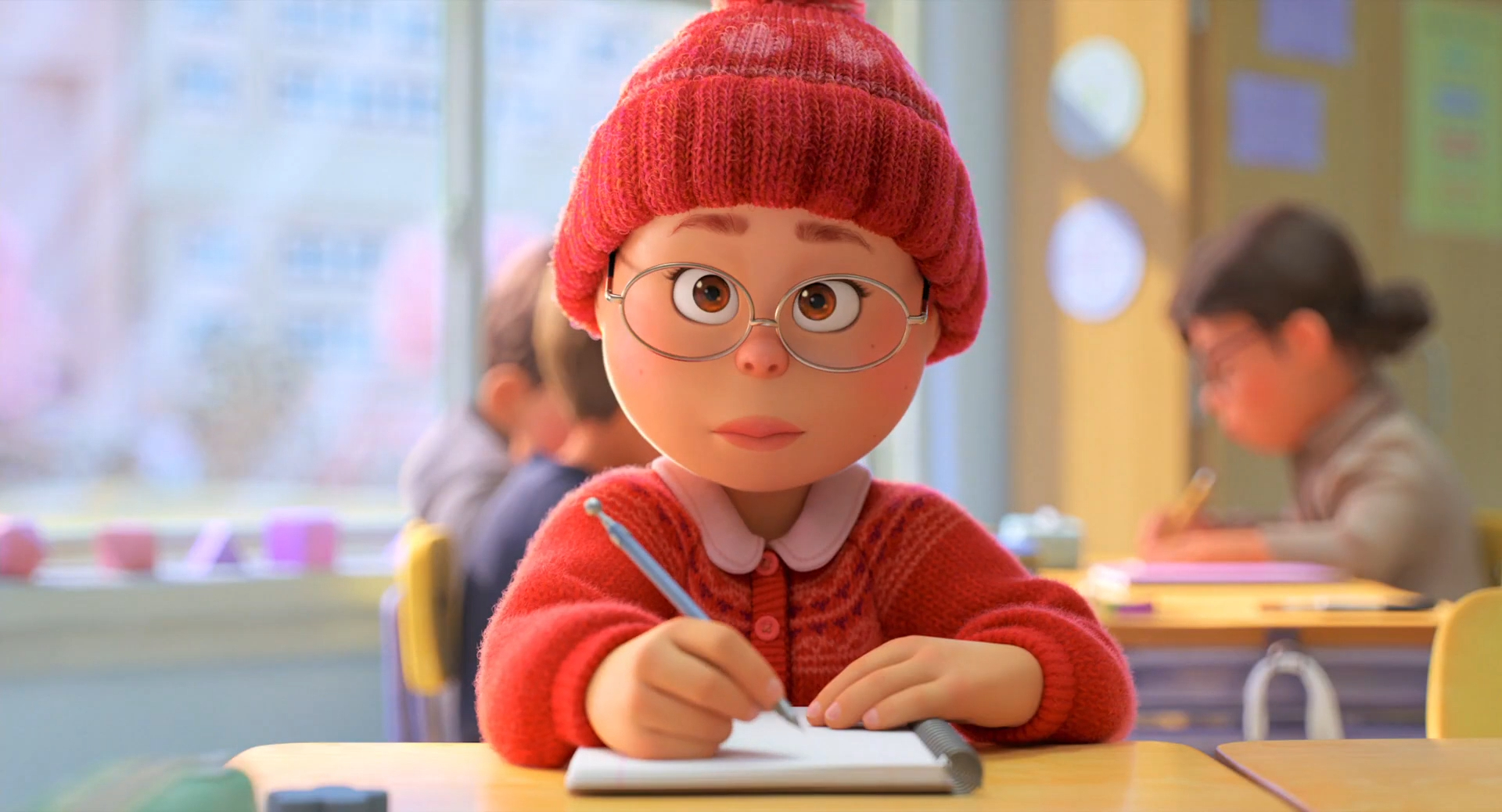Margo, the beloved character from "Despicable Me," is depicted sitting at a desk in what appears to be a cozy classroom setting. She wears her signature oval silver glasses and a charming red knit hat adorned with pink shapes at the top. Complementing her hat, she has on a red knit cardigan with a pink collar. Margo is captured holding a pencil in her right hand, poised to write in the notebook beneath her left hand. As she looks up from her notebook, she gazes directly into the camera, her slightly blushed cheeks and pink lips adding a touch of warmth to her expression.

In the softly blurred background, three other students are seated at a table, busy with their own tasks. A large window behind Margo allows sunlight to stream into the classroom, casting a gentle glow over the room. On the windowsill, various forms, including a pyramid and a cube, can be seen, adding an educational touch to the setting. The classroom is furnished with yellow chairs and light wooden desks, creating a vibrant yet inviting atmosphere.